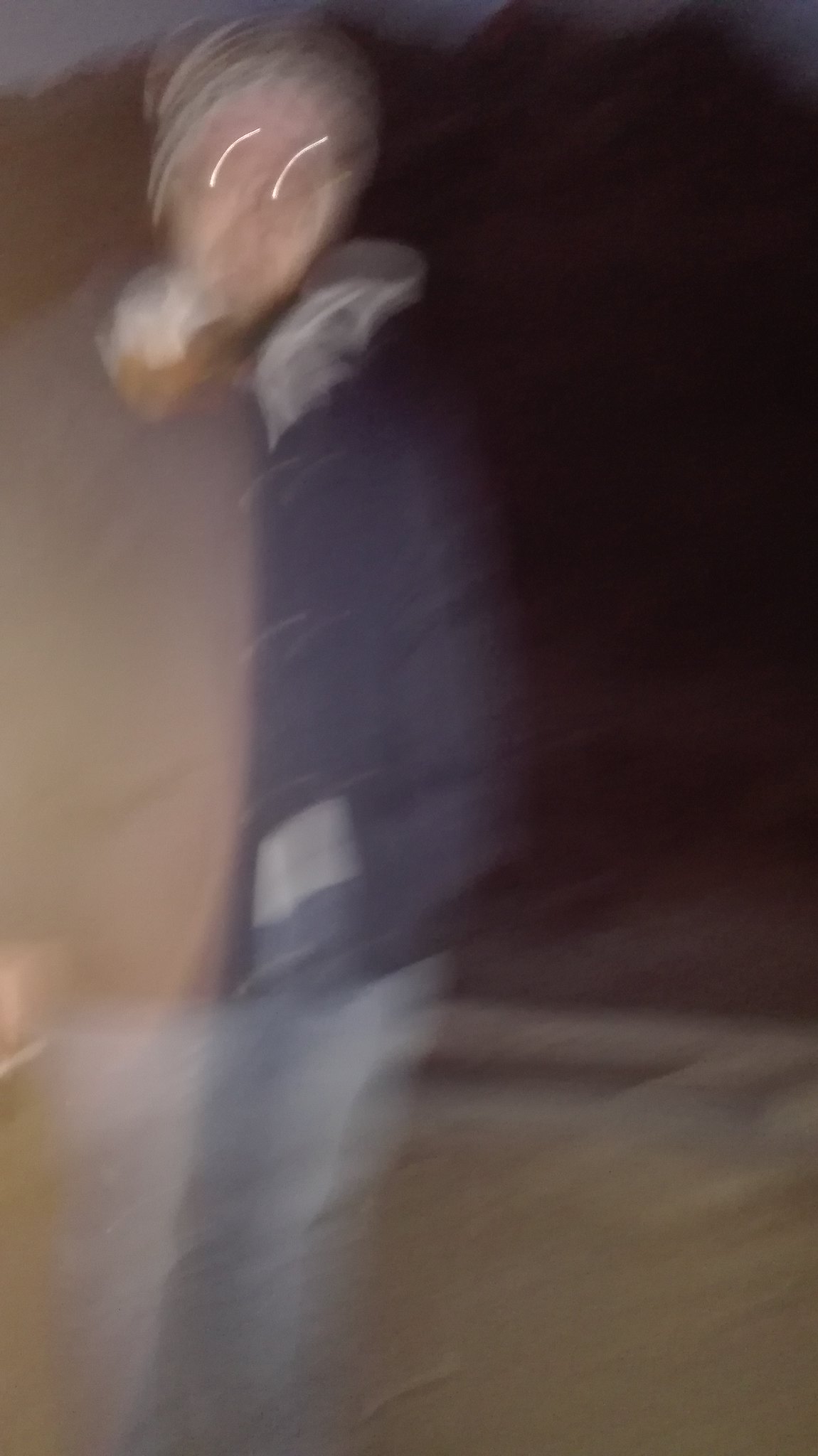This image captures a very blurry photograph of a person, likely a white male, that was taken quickly or with a moving camera, resulting in considerable distortion. The individual is wearing a grey beanie or snow cap that covers the ears, and a thick blue jacket, possibly with a fur collar near the head area. His pants appear to be light blue or dark-colored, with a strong indication that they are jeans. He is standing outside on a light brown ground, and the black sky behind suggests that the photo was taken at night, likely using a flash, as evidenced by the shiny, elongated white lines where his eyes should be, creating a somewhat distorted effect on his face.